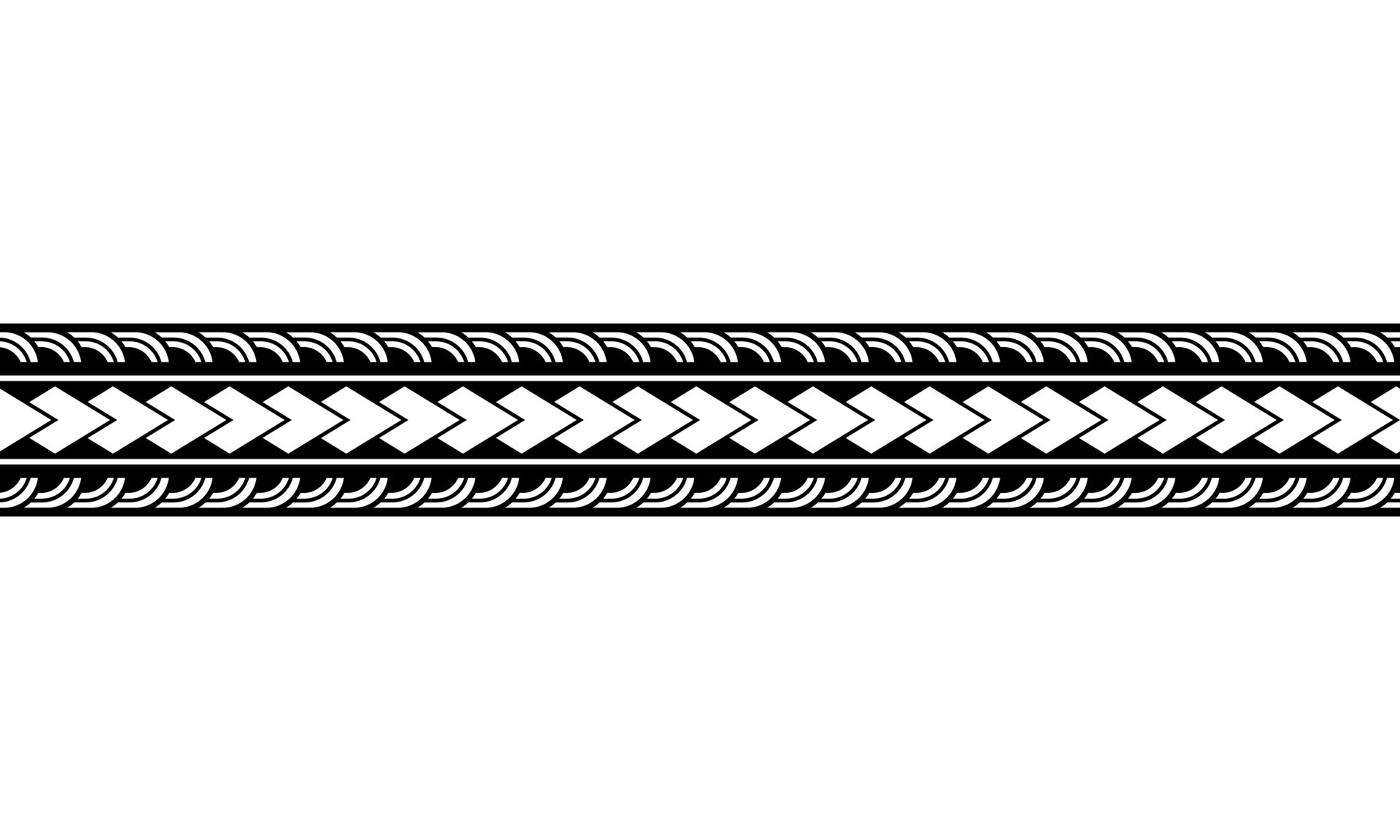The image features a detailed black-and-white illustrated pattern that extends horizontally from left to right across the center. The pattern, resembling a thin ribbon or a braided belt, is composed of three main horizontal sections laid out against a black background framed by a white backdrop above and below.

In the top section, there is a repeating border design consisting of sets of two curved lines—one smaller and one larger—that begin straight on the left and curve elegantly downward. These double lines repeat uniformly across the length of the ribbon, creating a visually engaging upper border.

The middle section is dominated by overlapping diamond shapes, which appear squat and horizontally stretched, with their tips pointing to the right. This creates a flowing, interconnected diamond pattern that aligns with the braided or woven feel of the entire design.

The bottom section mirrors the top, featuring the same pattern of double curved lines. However, in this section, the lines curve upward, effectively framing the central diamond pattern by balancing the curving motion from top to bottom, enhancing the overall symmetry and harmony of the pattern. The repetitive nature of these elements gives a sense of continuous movement across the design.